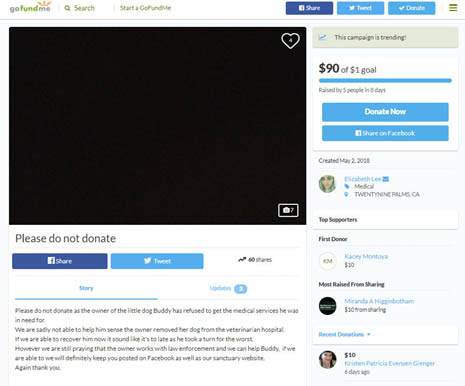**Caption:**
The image is a screenshot from a GoFundMe page. At the top left, the GoFundMe logo is clearly visible, along with the search bar and a "Start a GoFundMe" option. The page features a large black square, an unusual placeholder where a campaign’s main image typically appears, adorned only with a heart icon in the top right corner. Below the black square, the bold text reads "Please do not donate," emphasizing an urgent notice to potential contributors.

The page has generated some social media interest, with options to share the campaign via Facebook and Twitter, and it’s been shared 60 times. The accompanying narrative reveals a heartbreaking story: the campaign was originally set up for a dog named Buddy. Tragically, the owner refused essential medical services for Buddy and removed him from the veterinary hospital, resulting in Buddy's worsening condition. The plea now revolves around law enforcement intervention to possibly save Buddy, though the prognosis appears grim.

Despite the dire message, the campaign has managed to raise $90 from five donors, significantly surpassing its humble $1 goal. The campaign, which was trending, was created in May of 2018. Given the dated nature of the campaign, it is likely that Buddy is no longer alive. The image concludes with a list of donors and a few related pictures, marking the end of this sorrowful plea.